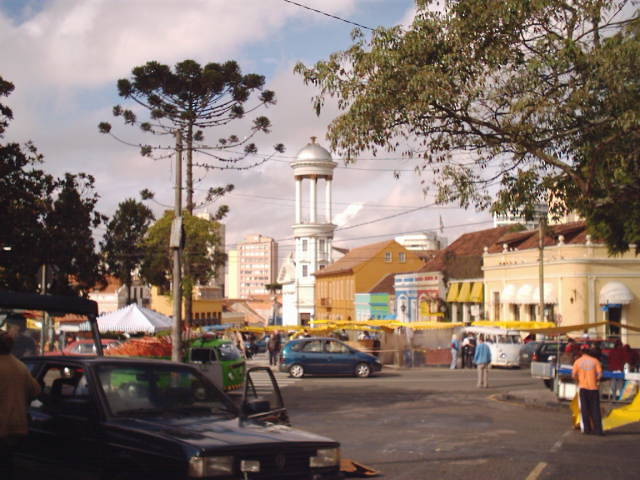A historic photograph captures a bustling European town center, likely from the 1990s, based on the style of cars and the people’s attire. The focal point of the image is a striking Romanesque-style pavilion, painted white and adorned with columns supporting a dome, standing approximately three to four stories tall. Surrounding this central structure are a variety of colorful shops and houses. The streets below are filled with pedestrians and a diverse array of vehicles, including sedans, blue vans, and a classic VW bus. In the distance, one can spot several high-rise buildings, suggesting a more urban area beyond the quaint center. The scene is set during a cloudy daytime, adding a nostalgic ambiance to the lively tableau.